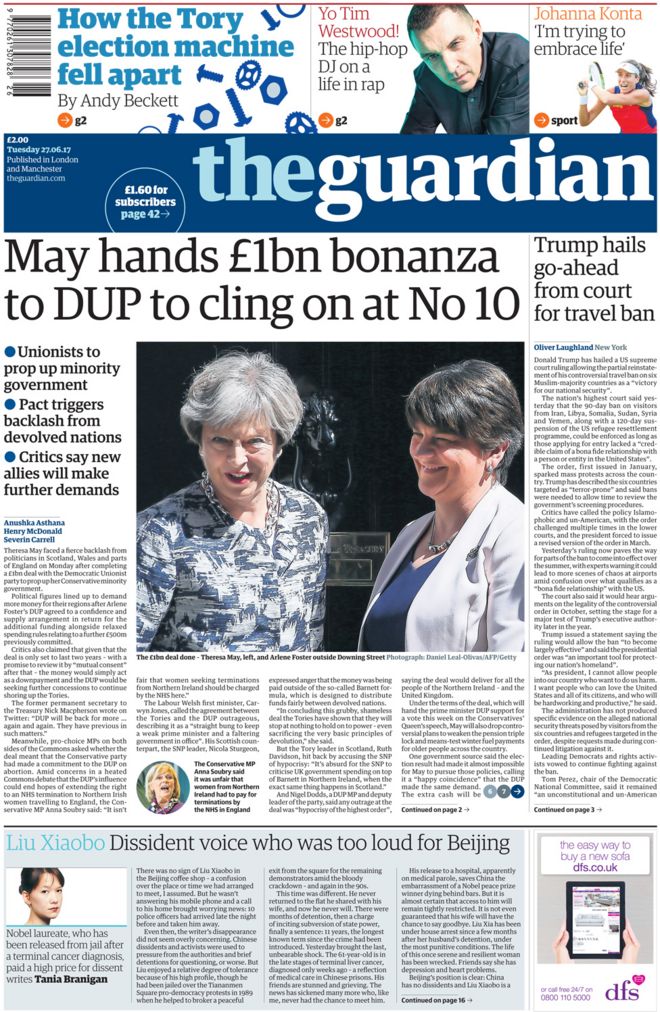This image captures the front page of The Guardian newspaper, prominently showing the barcode in the top left corner. The masthead indicates a publication date of Tuesday, June 27th, 2017, with a sale price of €2.00 or $1.60 for subscribers. This issue, published in London and Manchester, features several key articles and headlines across its layout.

At the top, the headline "How the Tory election machine fell apart" by Andy Beckett is featured in section G2, alongside "Yo! Tim Westwood, the hip hop DJ on a life in rap" also in G2. Another headline reads "Johanna Konta: ‘I’m trying to embrace life,'" positioned in the Sports section.

Prominent news articles include "May hands €1bn bonanza to DUP to cling on to No. 10," which is accompanied by images of Theresa May and Arlene Foster outside Downing Street. This piece discusses unionists propping up the minority government and includes details on the backlash from devolved nations and critics' concerns about further demands from new allies, continued on page two.

Another significant piece, "Trump hails go-ahead from court for travel ban," continues on page three. In the bottom left, there's a feature on Liu Xiaobo, described as a dissident voice too loud for Beijing. Nobel laureate Liu Xiaobo’s release from jail following a terminal cancer diagnosis is detailed by Tania Brannigan, emphasizing the high personal cost of his dissent.

In the bottom right corner, there is an advertisement for DFS, promoting "The easy way to buy a new sofa" with a visual of a tablet displaying their website, dfs.co.uk. The ad highlights their 24/7 customer service at 0800-110-5000. This detailed snapshot of The Guardian provides a comprehensive overview of its leading stories and features for the day.